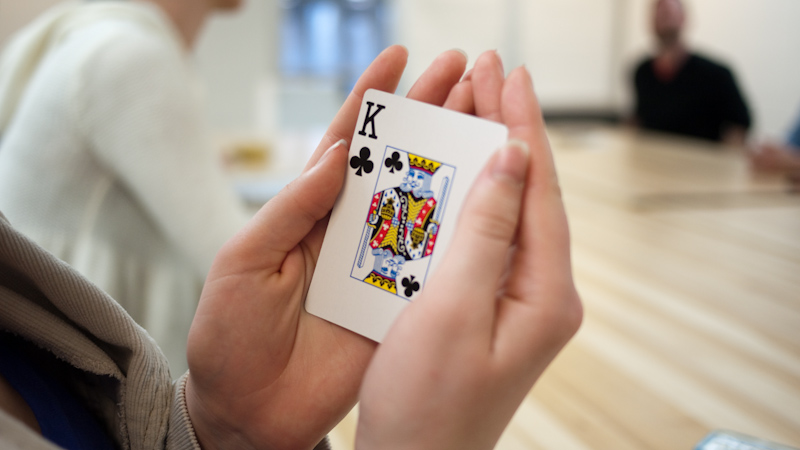In this image, a woman, identifiable by her longer fingernails and feminine appearance, is holding up a distinctive playing card. Both of her hands are carefully cupping the card, suggesting that she might be trying to conceal its value. The card is the King of Clubs, characterized by a white background with a minimalistic design: a thin blue square in the center, housing a small depiction of the king symbol and a 'K' in the top left corner with a club symbol directly below it. Unlike typical playing cards, the design is unusually sparse, occupying only the center portion of the card.

The background is blurry, but some details can be discerned. To her right, a man wearing a black shirt, who appears to be of African descent, is partially visible. On her left, another individual wears a white long-sleeve shirt. Although the rest of the scene is unclear, it appears they are gathered around a large table, possibly indicating a commercial or social setting. The person holding the camera seems to be someone else as both of the woman's hands are occupied with the card. The overall scene suggests they might be engaged in a card game, with the woman keenly shielding her cards while possibly posing for a picture taken by a friend.